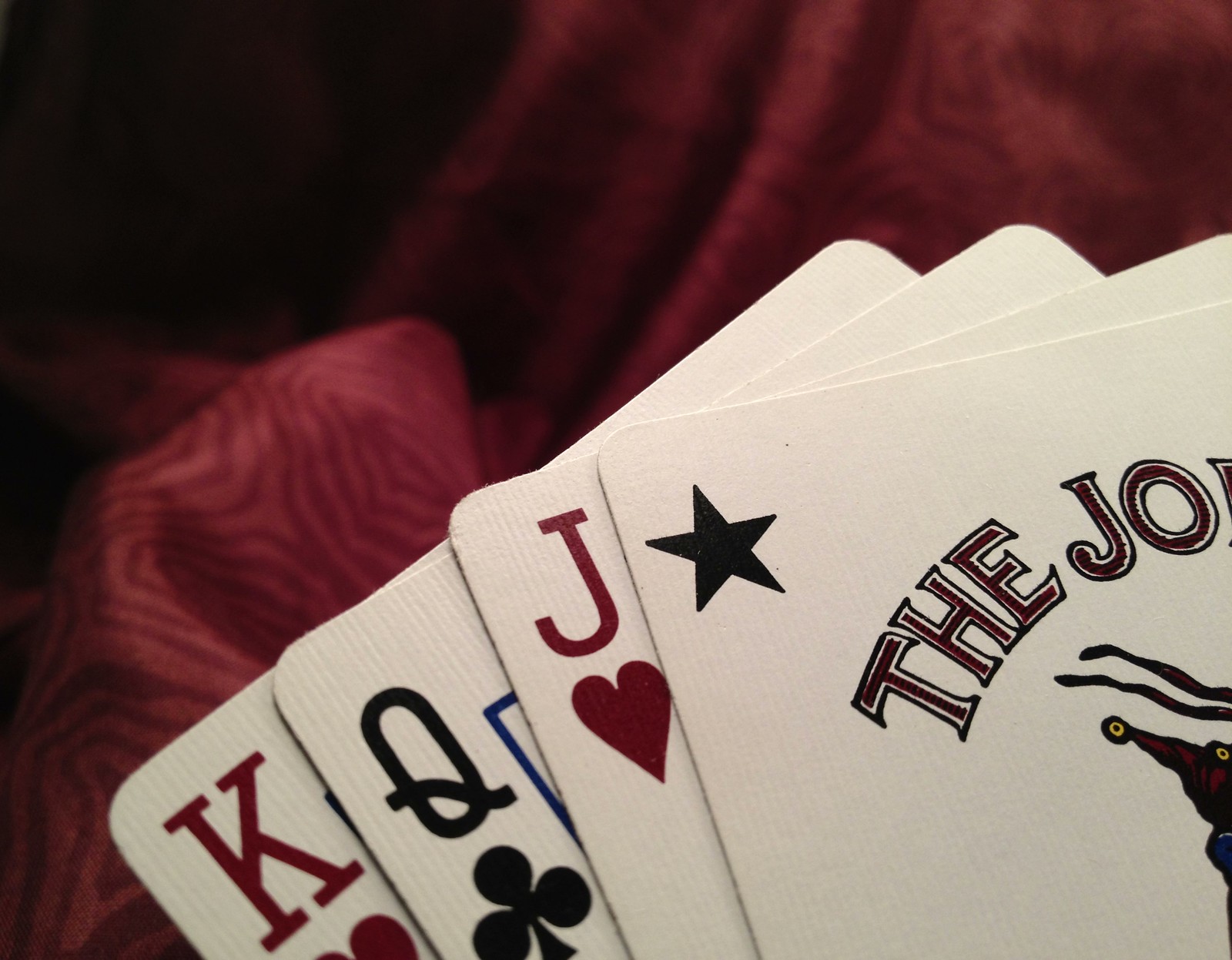In this image, we observe an arrangement of four cards, fanned out as if held in a hand during a card game. The foremost card is the Joker, identifiable by a black star in the top left corner and the partially visible word "Joker" in the bottom right corner. Following the Joker, the succeeding card is the Jack of Hearts, only partially visible with the "J" and the heart symbol lightly showing. The third card in the sequence is the Queen of Clubs, discernible by the letter "Q" and a small portion of the club symbol. Lastly, the fourth card appears to be the King of Hearts, mainly exposing the "K" and a slight indication of the heart symbol. These cards are set against a background of a luxurious red blanket, embellished with an intricate pattern, enhancing the overall rich and refined aesthetic of the scene.